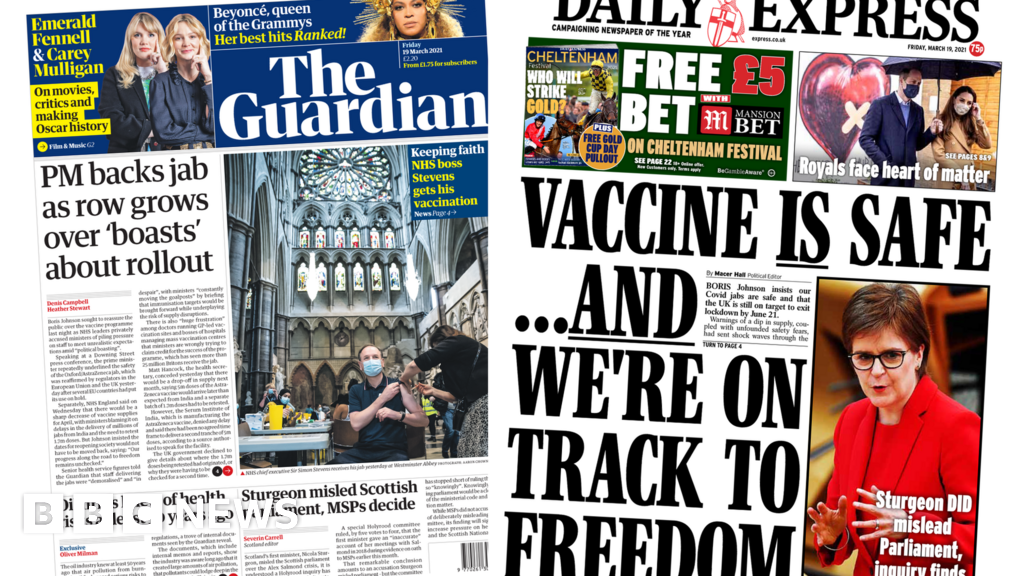In the image, we see a couple of pages from newspapers and magazines. On the right, there is a page from the Daily Express, which appears to be the front cover. This cover prominently features an article on the Royal Family, titled "Royals Face, Hearts of Matter." The image shows Prince William and Princess Kate walking out of what seems to be a heart hospital or heart charity foundation. The weather is rainy, as evidenced by the black umbrella they are carrying, and Prince William is wearing a black mask. The major headline on this front cover reads, "Vaccine is Safe and We're on Track to Freedom," indicating a significant update on the COVID-19 vaccine progress. Additionally, there is a photograph of an older woman in a red suit, possibly a notable figure, contributing to the article themes.

On the left side of the image, there is a page from The Guardian, which is likely an inner page rather than the front cover, given the large amount of text. The main headline on this page states, "Prime Minister backs jab as row grows over boasts about rollouts." This page includes a stock photo depicting COVID-19 testing being conducted inside a grand cathedral, adding visual context to the text-heavy article.